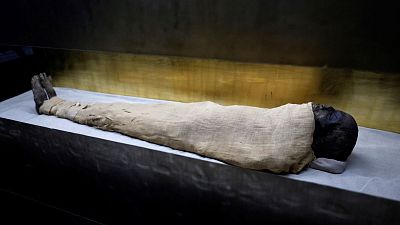This photograph captures a somber scene of a mummified body, presumably of a black individual, resting on a white pedestal or a wooden coffin constructed from a hollowed-out log. The mummy is tightly wrapped in a burlap sack-like material that covers the entire body except for the head and feet. The head, although dark-skinned and marked by time, retains distinct facial features such as the eyes and nose, and rests on a small mat or pillow. The feet, starting to shrivel into bone, starkly protrude from the wrapping. The overall setting is dimly lit, casting a mix of shadows and reflections that interplay with the gold background and a reflective horn positioned behind the body, enhancing the solemn and eerie atmosphere of the scene.